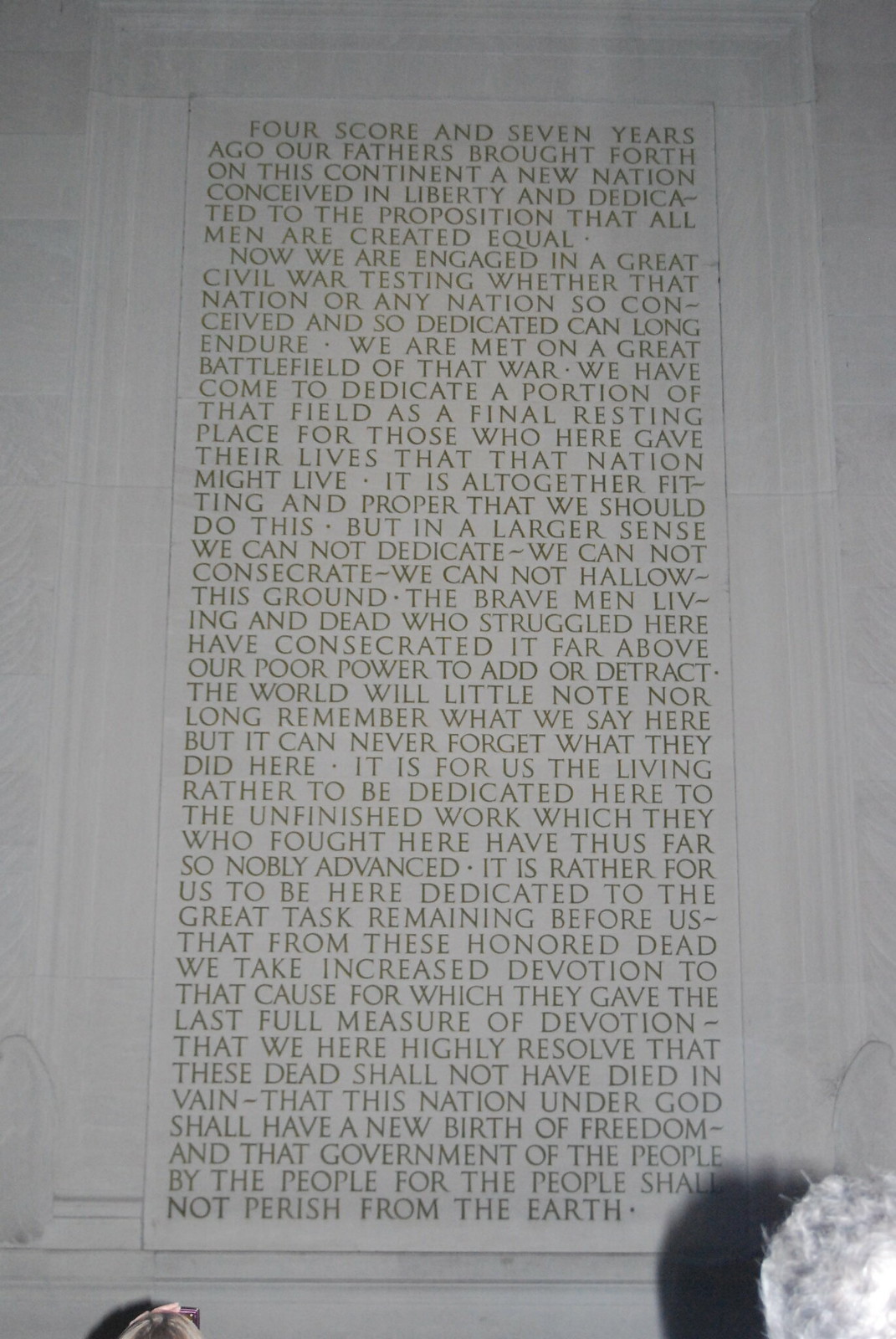The photograph shows the Gettysburg Address etched in all-capital letters onto a large, gray marble wall, part of the Lincoln Memorial in Washington, D.C. The inscription is seamlessly embedded into the wall, appearing almost like a goldish-brown scroll laid out for visitors to read. The historic speech, which starts with "Four score and seven years ago" and concludes with "the government of the people, by the people, for the people, shall not perish from the earth," is prominently displayed in a rectangular format, likely in a Times New Roman font. In the foreground, the tops of two heads can be seen; on the lower right, an elderly person with a full head of gray, curly hair, and on the lower left, a young girl raising a cell phone to capture the monumental text.